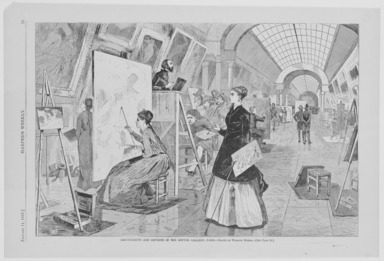The detailed black-and-white illustration, rendered in an 18th-century style using pen and ink, depicts a lively indoor scene likely set in a museum or an art studio. Dominating the foreground are two women: one seated on a stool, immersed in painting a large canvas, while the other, dressed in a long dark frock or coat, carefully observes her work. This central duo is flanked by additional figures who are also engaged in artistic activities, painting on canvases positioned throughout the spacious room. The room itself is striking, featuring an arch-shaped ceiling with glass skylights that allow natural light to pour in, illuminating the creative environment. In the upper left of the image, on a raised platform, a bearded gentleman holding a book appears to be overseeing the entire scene, possibly conducting what seems to be an art auction, given the gestures and interactions of other figures in the vicinity. The walls are adorned with numerous framed artworks, enhancing the atmosphere of this meticulously designed interior space.